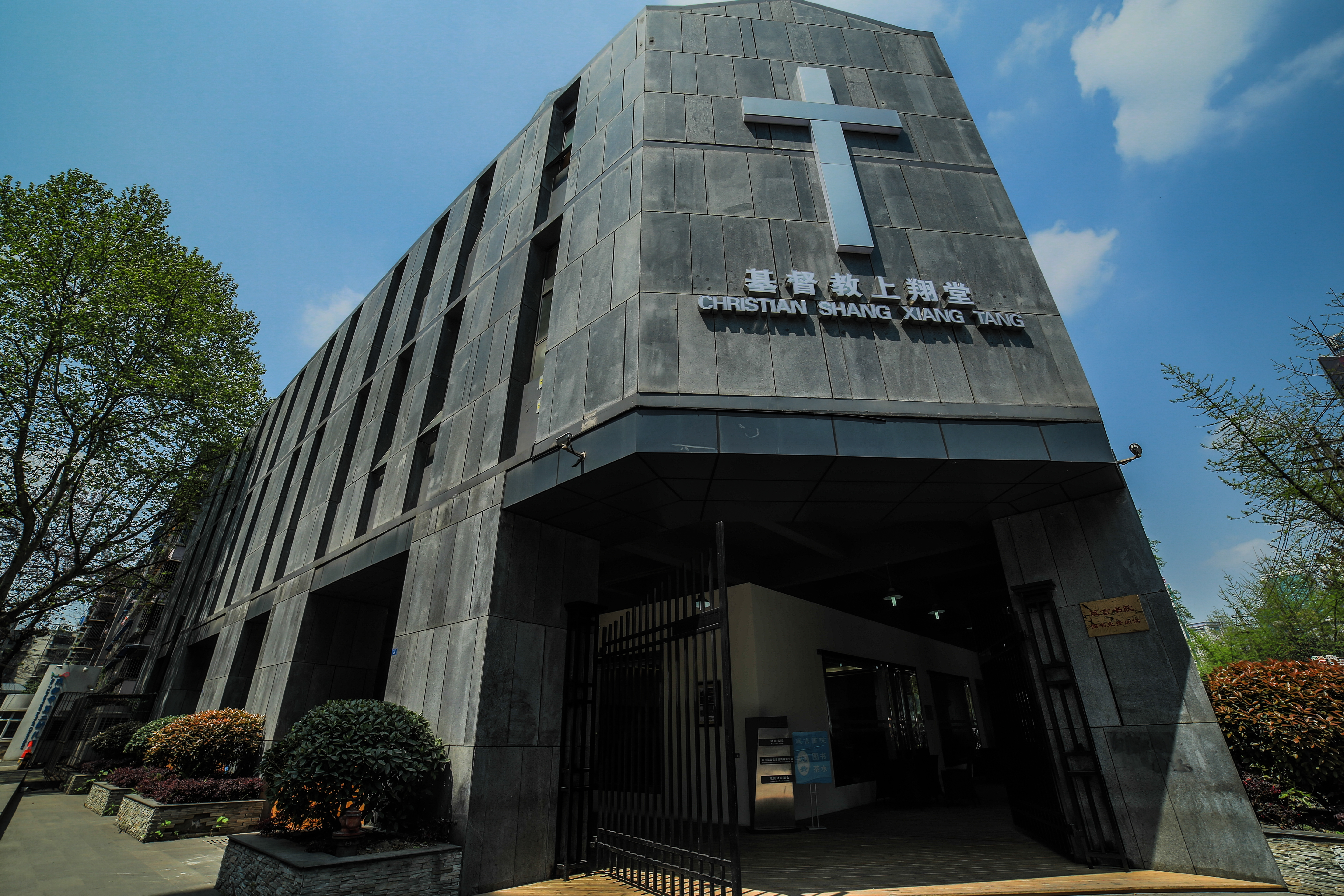The image depicts a modern, sizeable church building named "Christian Sheng Yangtang." The structure, composed of dark gray and black concrete and grayish brick, stands approximately four stories tall with a distinctive rectangular design. A prominent silver cross is affixed in front of the building, just above the church's name, which is displayed in both Chinese characters and English text. The text and cross are three-dimensional, adding depth to the façade.

In front of the church, there is a black wrought iron gate, currently half-open, inviting entrance. On both sides of the building, lush greenery is present, including bushes and trees, with larger stone planters positioned on the left side. The trees and bushes add a touch of nature to the otherwise modern and clean design. The sky above is a clear blue with visible clouds, indicating a sunny day. There are no people in the image, and the scene is devoid of activity. The photograph is of high quality and offers clear details of the architectural elements and surroundings.